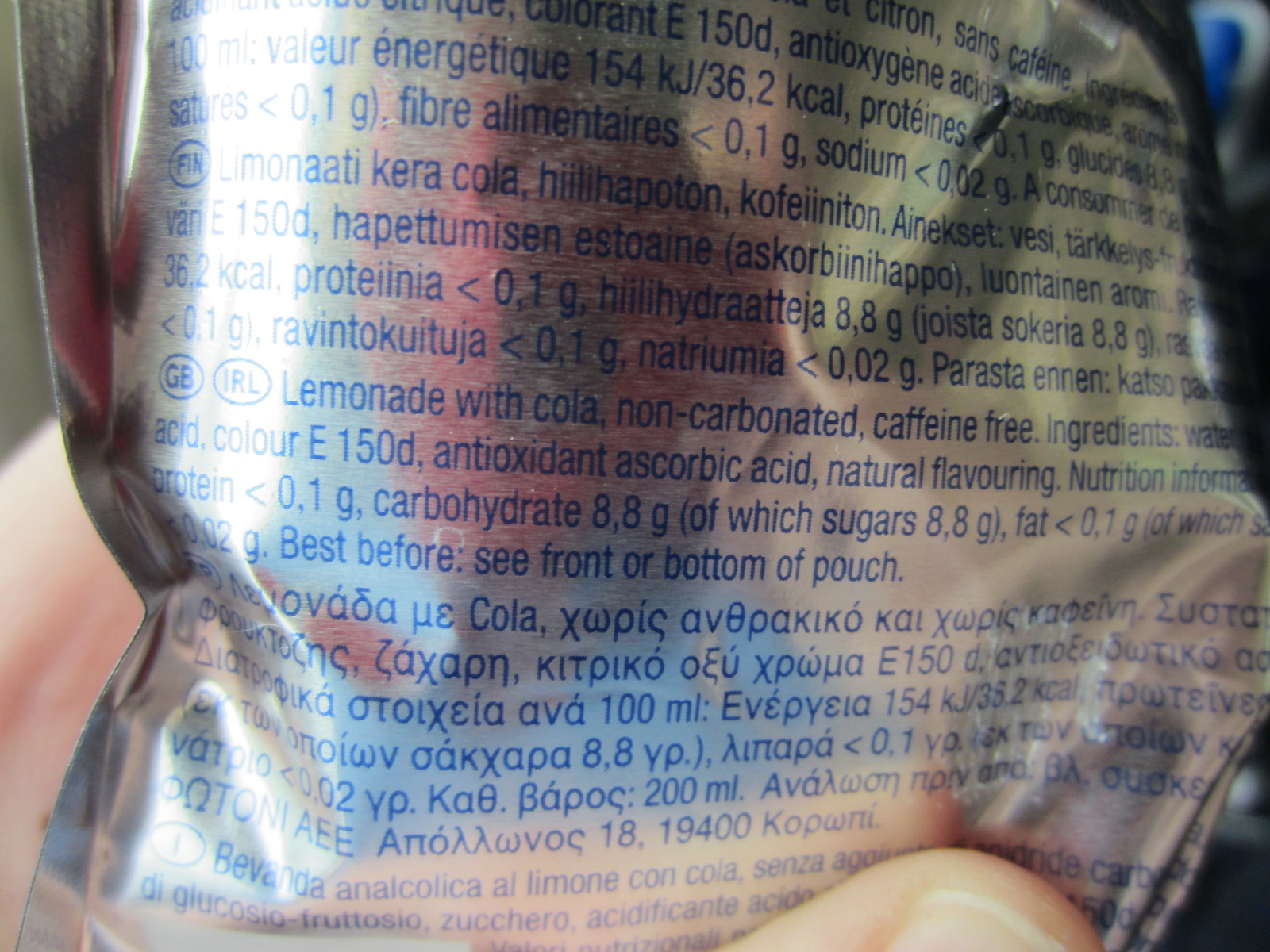This close-up image captures a shiny silver package, prominently held by a hand with the thumb and a few fingers clearly visible. The package features a multilingual label, with the English section describing the contents as "lemonade with cola, non-carbonated, caffeine-free." The ingredients listed are water, acid, coloring, ascorbic acid, and natural flavoring. Additionally, it provides some nutritional information and states "Best before: see front or bottom of pouch." Above and below the English text are sections in multiple other languages, reflecting the product's international market appeal.